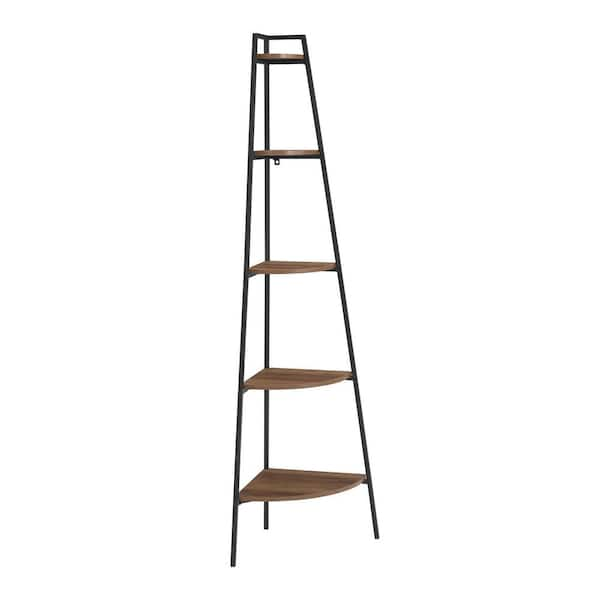The image features a tall, six to seven-foot corner shelf designed for displaying and storing items. The shelf structure is supported by three black metal poles arranged in a triangular formation, with the central pole ascending straight up while the left and right poles slope inward. The five tiers of shelves, crafted from dark brown wood, decrease in size as they ascend, with the largest shelf at the base and progressively smaller ones above it. Each shelf is triangular, fitting neatly into a corner space. The entire unit is set against a plain white background, emphasizing its minimalist and functional design. The shelf is empty, showcasing its clean, simple lines and modern aesthetic.